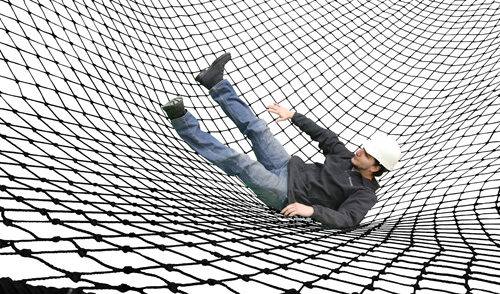The image depicts a man laying on his back in the middle of a large black net, as if he has just fallen into it from a height. The net, which appears to be a safety net likely used in a training course for utility workers or similar professionals, spans the entire frame. The man is wearing a white hard hat, a black three-quarter zip jacket with white text on the top left, light blue jeans, and steel-toed black boots. His legs are raised, and his arms are extended outward. The man has some facial hair on the left side of his face, adding more detail to his appearance. This scene suggests a practical exercise in safety protocols for high-risk jobs involving ladders or elevated equipment. For more information, visit www.FEMA.gov.